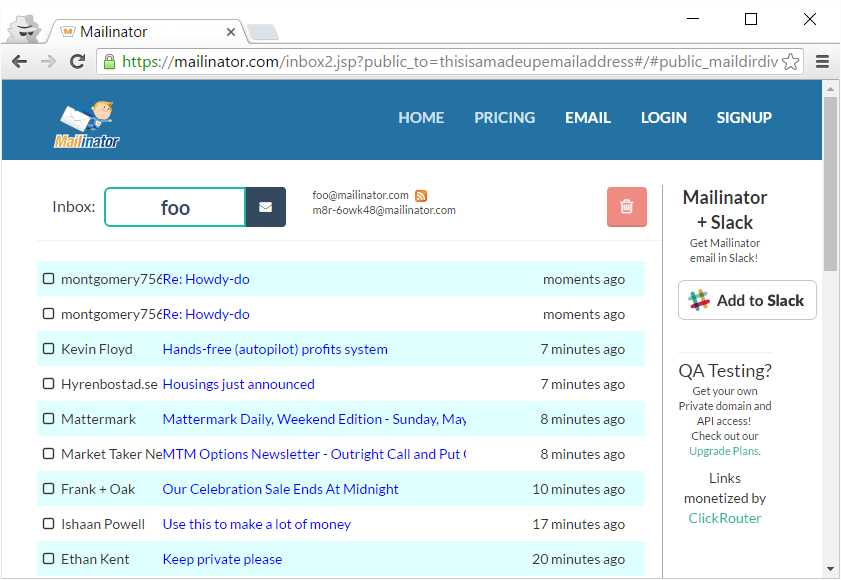This image captures a screenshot of the Mailinator website. The URL "https://mailinator.com" is clearly visible in the browser's address bar, ensuring the site’s secure connection. The Mailinator logo, featuring a superhero flying with an envelope, is prominently displayed. Below this logo, the inbox labeled "foo" (F-O-O) is shown, with the address "foo@mailinator.com" beside it.

The main section of the page displays a series of emails in the inbox, starting with "Montgomery 756" with a subject line of "RE: howdy do," which is repeated for the following email. Other notable subject lines include "hands-free autopilot profit system," "housing just announced," "Mattermark daily," "weekend edition, Sunday, May," "use this to make a lot of money," and "keep private, please." The emails are listed in succession down the page. Additionally, the sides of the page contain clickable ads, adding some interactive elements to the site’s layout.